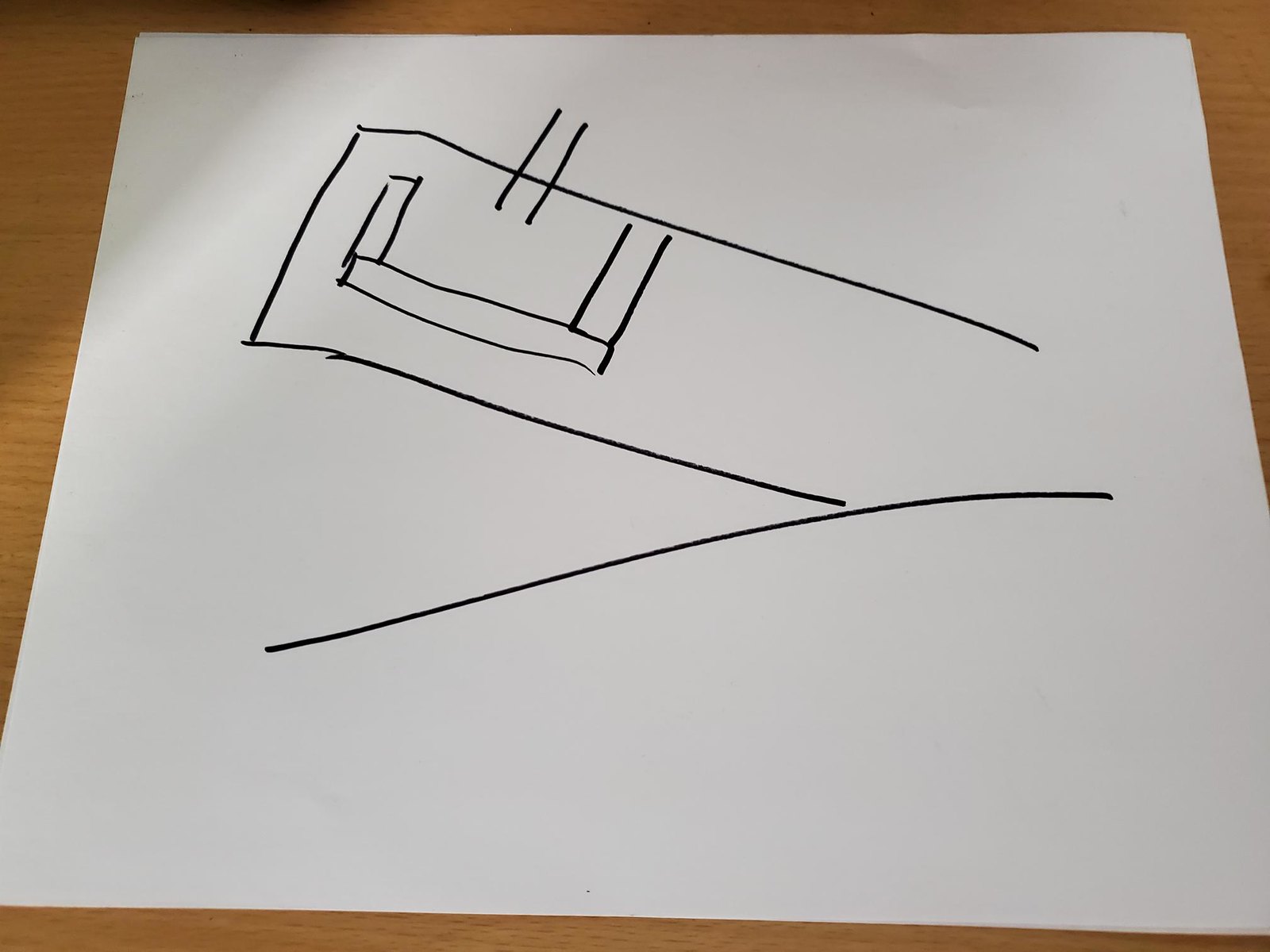The image features two sheets of white paper resting on a wood grain surface. The second sheet is partially visible, with its edges peeking out from beneath the top sheet in both the upper left and upper right corners. The top sheet showcases a rudimentary sketch in black felt-tip pen, reminiscent of an architectural drawing. This basic design includes a slanted, curved line at the bottom, likely representing the terrain or horizon. In the center of the paper, a large, tilted rectangle appears to delineate the walls of a room or living space. Within this larger rectangle are three smaller, connected rectangles, suggesting elements like furniture—a table, perhaps—and a walkway. Two intersecting lines at the perimeter of the larger rectangle seem to illustrate a window, doorway, or another form of access.